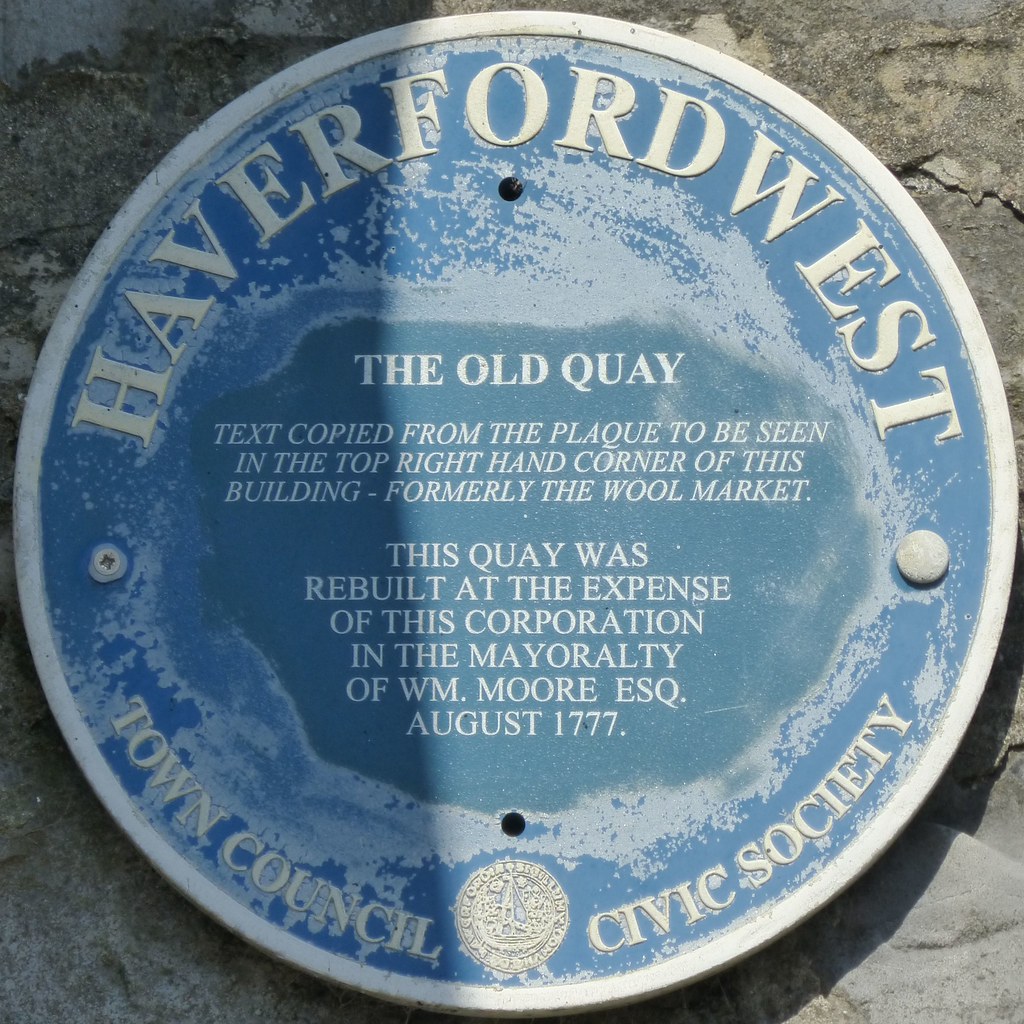This image is a color photograph of an outdoor circular plaque affixed to a stone or concrete gray wall. The plaque, which appears to be metal and blue in color with faded paint, features silver text detailing historical information. Around the top, the plaque is labeled "Haverford West," and around the bottom, it reads "Town Council Civic Society," with a small emblem situated between "Council" and "Civic."

In the center of the plaque, in bold white font, it reads "The Old Quay." Below, still in capital letters, the text continues: "Text copied from the plaque to be seen in the top right-hand corner of this building, formerly the Wool Market. This quay was rebuilt at the expense of this corporation in the mayoralty of William Moore Esquire, August 1777." 

The overall design presents a detailed historical record of the location, marked by clear but time-worn text on a background that speaks to its long-standing presence.